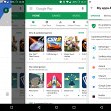The image depicts a small and blurry rendering of a digital device screen displaying the Google Play Store, which could be a computer, tablet, or phone screen. Dominating the top part of the screen is a green banner with a white rectangle at its center, prominently featuring the text "Google Play." In the upper left-hand corner, there is a medium blue triangle adding a hint of color contrast.

Directly below the Google Play banner, there are several indistinct options, and to the right side, there is a menu, though the text is too blurry to read. The screen features six squares arranged in two horizontal rows, each representing different items, likely games.

In the first row, the central square appears to depict a game involving a car, with the game titles printed underneath in black text, although they are illegible due to the blurriness. The second row also contains three squares; the middle one is red and seems to feature an image of a rocket. At the very bottom of the screen, a thin black rectangle forms the footer of the display.